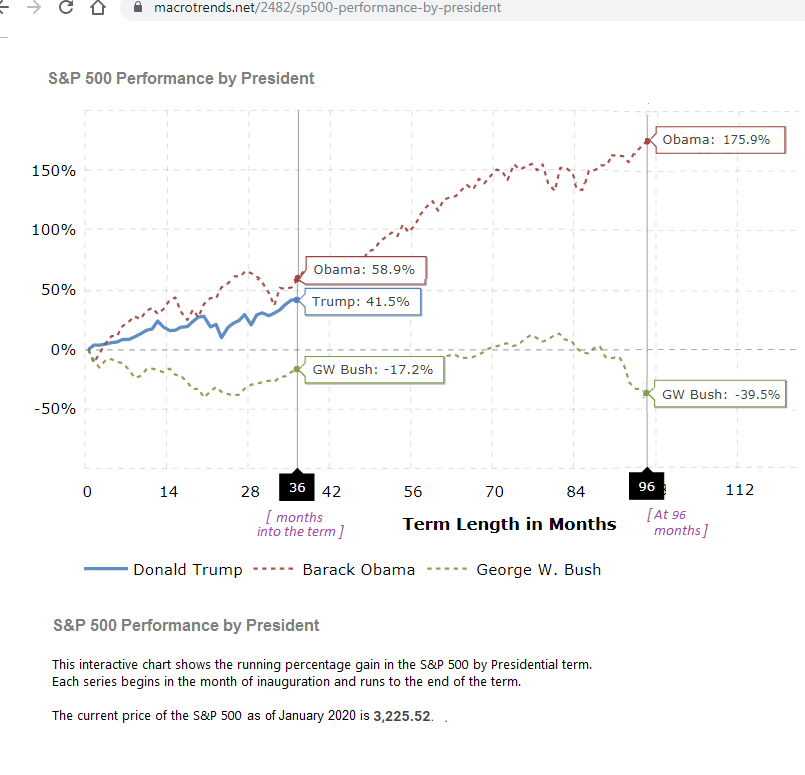The image features a detailed line graph titled "S&P 500 Performance by President," displaying the running percentage gains in the S&P 500 index during the presidential terms of Barack Obama, Donald Trump, and George W. Bush. The graph compares three lines, each representing a different president: a red dashed line for Obama, a blue line for Trump, and a green dashed line for Bush. 

The y-axis of the graph ranges from -50% to 150% in 50% increments, while the x-axis represents the term length in months, extending from 0 to 112 months. Obama's performance is depicted with notable highlights: 58.9% at 36 months and 175.9% at 96 months. Trump's performance shows a 41.5% gain at 36 months. In contrast, Bush's presidency is marked by negative performance, with a -17.2% at 36 months and a -39.5% at 96 months. 

The current price of the S&P 500 as of January 2020 is noted as 3225.52. This interactive chart provides a clear visual representation of the fluctuations in the S&P 500 index corresponding to the tenures of the three presidents, starting from their respective inaugurations to the end of their terms.